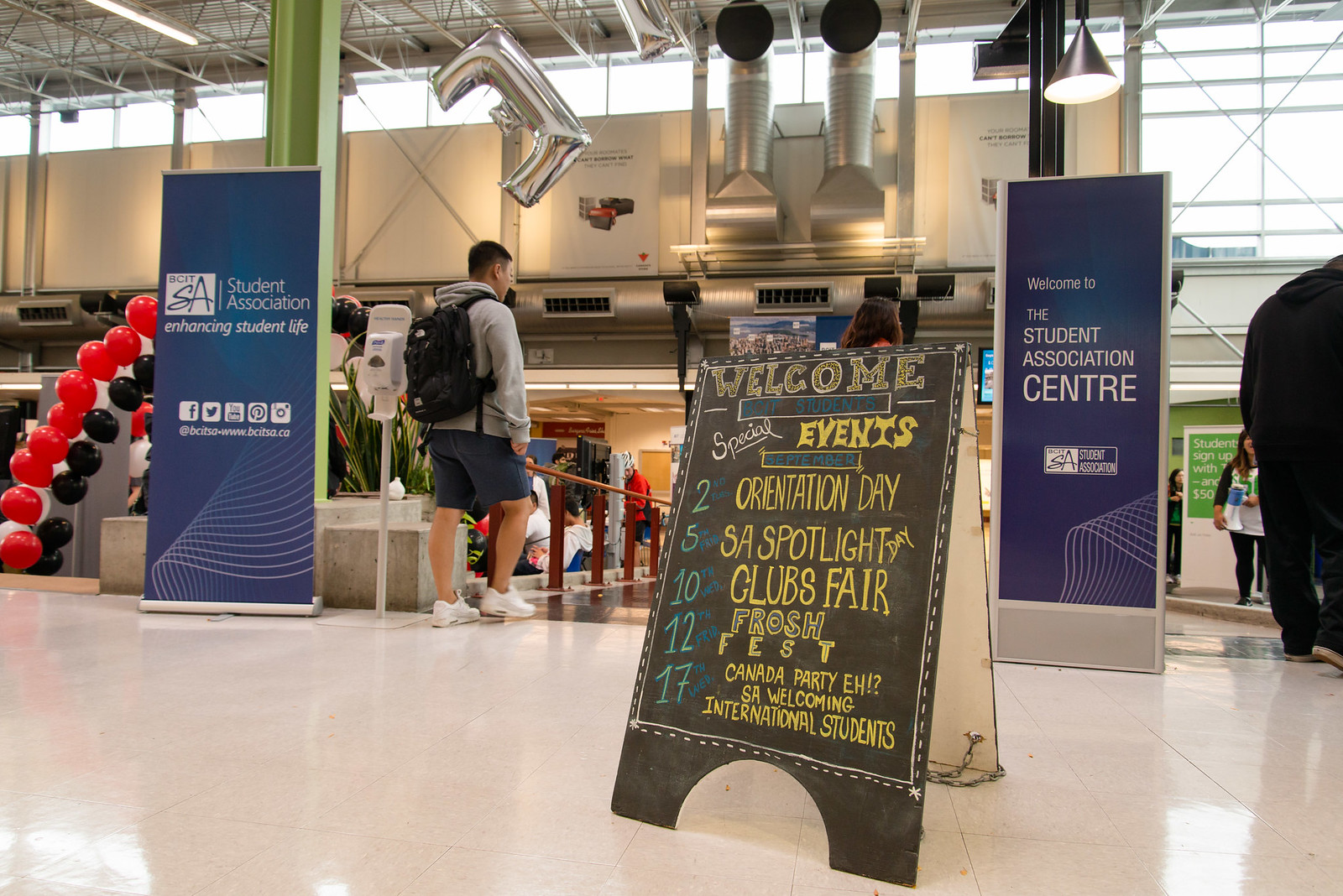The image captures the interior of a large, institutional gathering space reminiscent of a student center or event hall, similar to an airport terminal. The floor, situated toward the bottom of the image, is white tile with a glossy finish. At the center, there is a prominent black A-frame chalkboard sign with yellow letters that reads "Welcome BCIT Students" and lists various events including Orientation Day on September 2nd, SA Spotlight on the 5th, Clubs Fair on the 10th, Frosh Fest on the 12th, and Canada Party A on the 17th for welcoming international students.

On either side of the area, two vertical rectangular banners in dark blue with white text announce "Student Association Center" and "Student Association Enhancing Student Life." On the left side, a hand sanitizer station and a set of red and blue balloons draw attention. Further to the right, a young man is approaching a wooden handrail leading to a ramp. He is dressed in a gray hoodie, blue shorts, white sneakers, and a black backpack. In the distance, large windows let in ample natural light, brightening the space and highlighting additional details like a "take a number" meter and a clothing retail area on the left side of the walkway, just before the ramp.